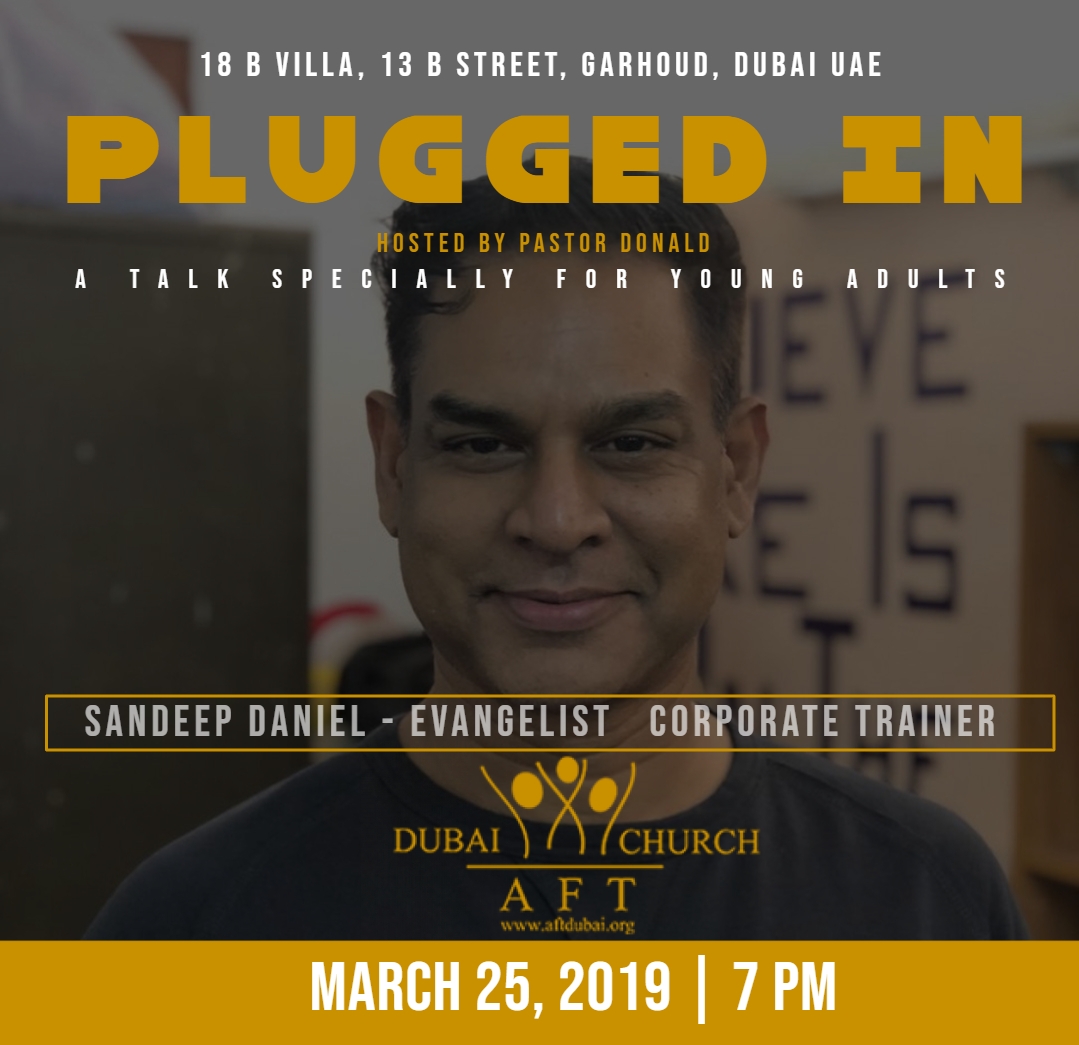The image is an advertisement flyer showcasing a church event featuring a speaker. Prominently displayed at the top is the location: "18B Villa, 13B Street, Garhoud, Dubai, UAE." The headline "Plugged In" is written in large, golden-yellow letters, followed by smaller gold text that reads "Hosted by Pastor Donald." The flyer describes the event as "A Talk Specially for Young Adults." 

The central figure in the flyer is an Indian male, likely in his 30s or early 40s, with short black hair, dark eyes, and light pink lips. He's smiling subtly and wearing a black t-shirt, looking directly at the camera with a proud or content expression. His name, "Sandeep Daniel – Evangelist, Corporate Trainer," is written in white text within a long, thin golden-yellow box placed near his chin. 

Below his name, the logo "Dubai Church AFT" is displayed, along with the website "www.aftdubai.org." At the very bottom, a golden-yellow bar features the event's date and time: "March 25th, 2019, 7 p.m."